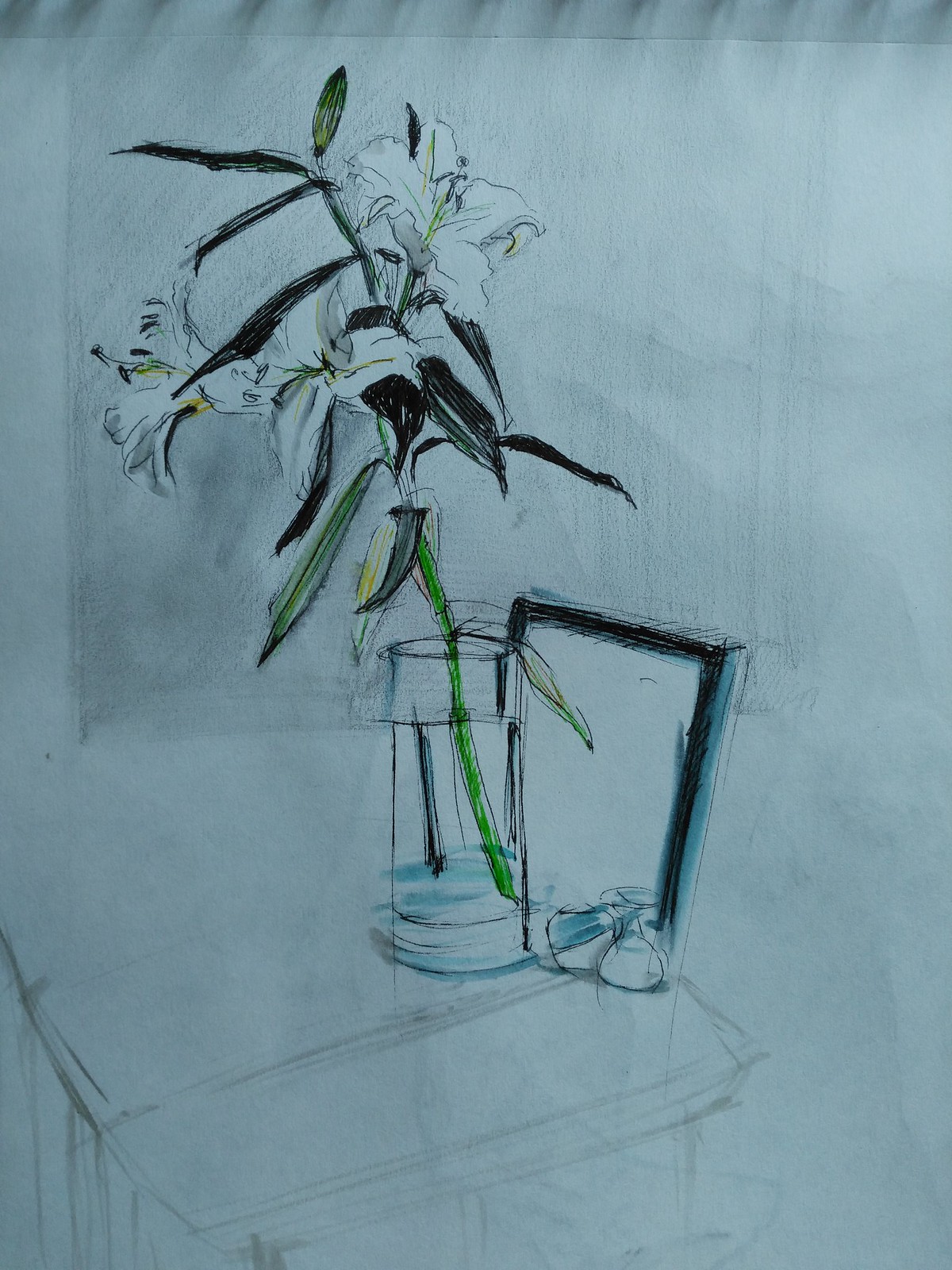The image is a detailed ink and watercolor sketch showcasing a white flower, possibly a lily, in a clear, tube-like vase filled with water that is subtly shaded blue. The stem and some leaves of the flower are painted green, while other leaves exhibit black hues. The vase is positioned on a desk, alongside what appears to be a partially drawn book. The background features vertical ruffles or shadowy lines suggestive of a window, with the overall composition remaining largely in pencil, giving a partially completed appearance. Small objects are placed near the vase, enhancing the desk's ambiance.